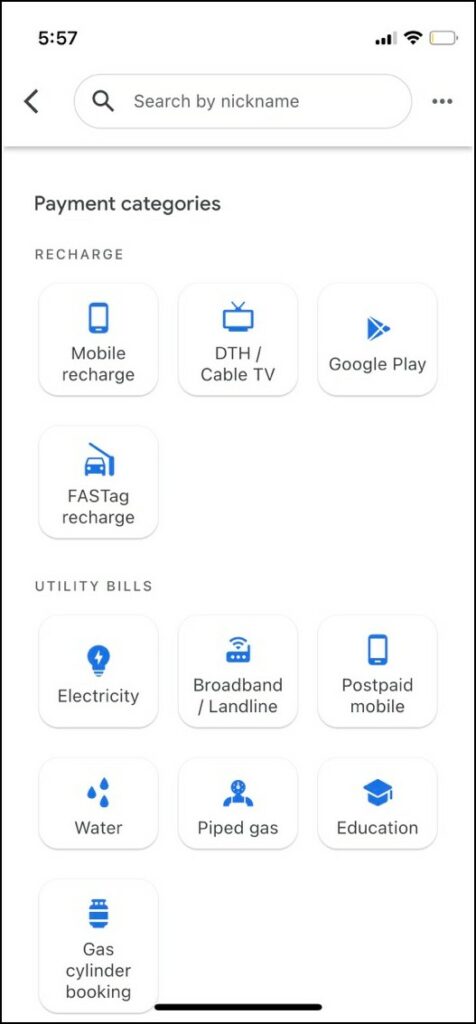Screenshot from my phone taken at 5:57 PM, showcasing a nearly drained battery, 3 bars of signal, and Wi-Fi connected. At the top of the screen, there is a search bar labeled "Search by nickname" with a back button to the left and a context menu with three dots on the right. Below this is a white background with black lettering, displaying various payment categories organized under different sections.

The categories listed includerecharge options for mobile and DTH/cable TV, Google Play, and FASTag recharge. Under utility bills, the options are electricity (represented by a light bulb icon), broadband/landline, postpaid mobile, water (depicted by three drops of water), piped gas, education (illustrated with a graduation cap), and gas cylinder booking. The icons for each category are in blue. Despite being unsure of the financial application's origin, the detailed icons and categories suggest it's a comprehensive financial tracker.